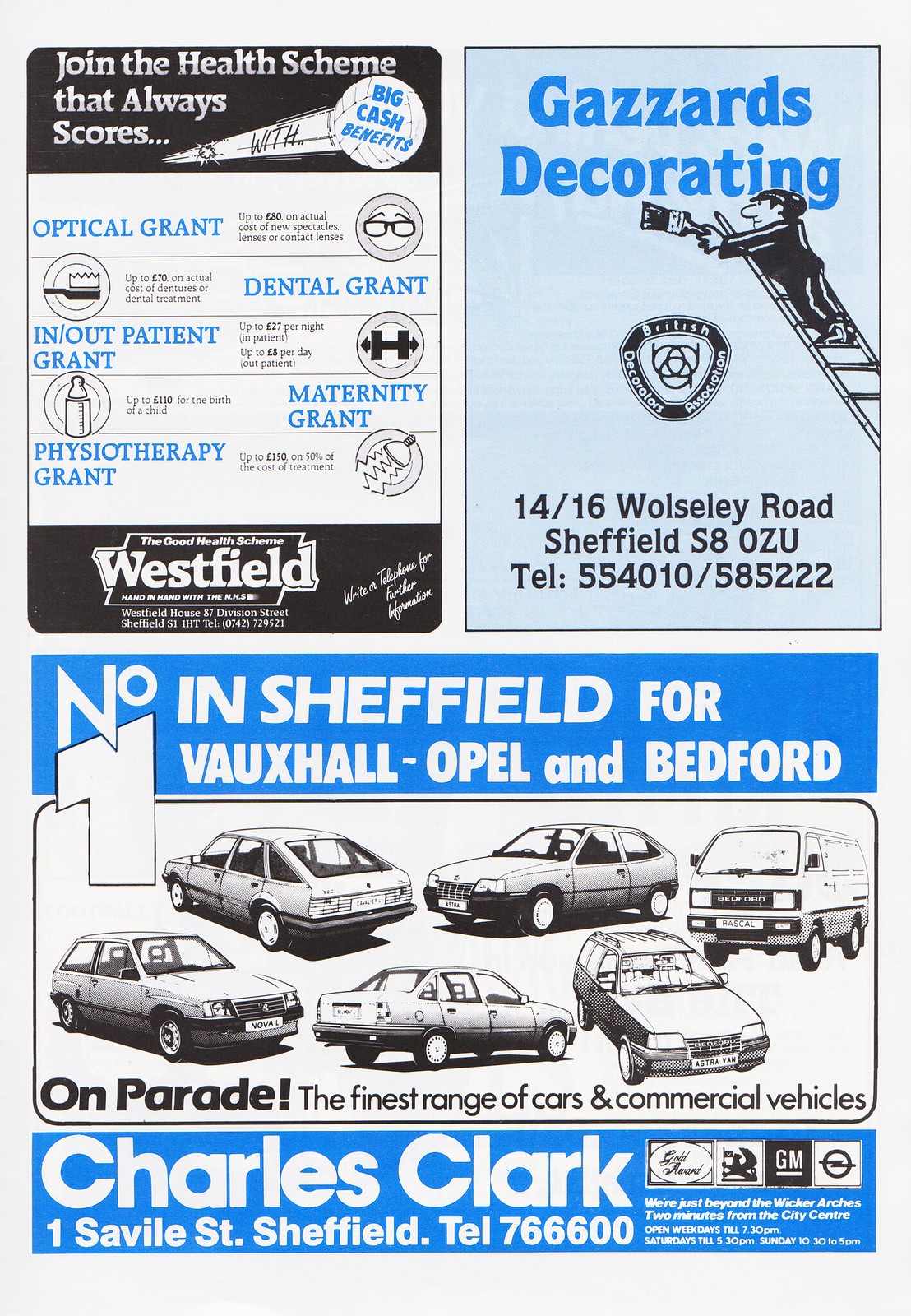The image showcases a trio of vintage advertisements, stacked in three rows within a rectangular frame. The top left advertisement, with a distinctive black border and white text, promotes a health scheme through Westfield, featuring benefits such as optical grants, dental grants, in and outpatient grants, maternity grants, and psychotherapy grants. The middle section of this ad emphasizes "Big Cash Benefits" within a circular design. On the top right, the ad for Gazzard’s Decorating displays a monochromatic cartoon of a man on a ladder holding a paintbrush, along with their address at 14/16 Rolesley Road, Sheffield, and contact number 54010/585222. Highlighted in blue, it also mentions the British Decorators Association. The bottom ad, centered around the slogan "Number One in Sheffield for Vauxhall, Opel, and Bedford," features six different cars in a parade format under the tagline "The Finest Range of Cars and Commercial Vehicles." This advertisement is attributed to Charles Clark, located at 1 Savelle Street, Sheffield, with a contact number of 766-600.